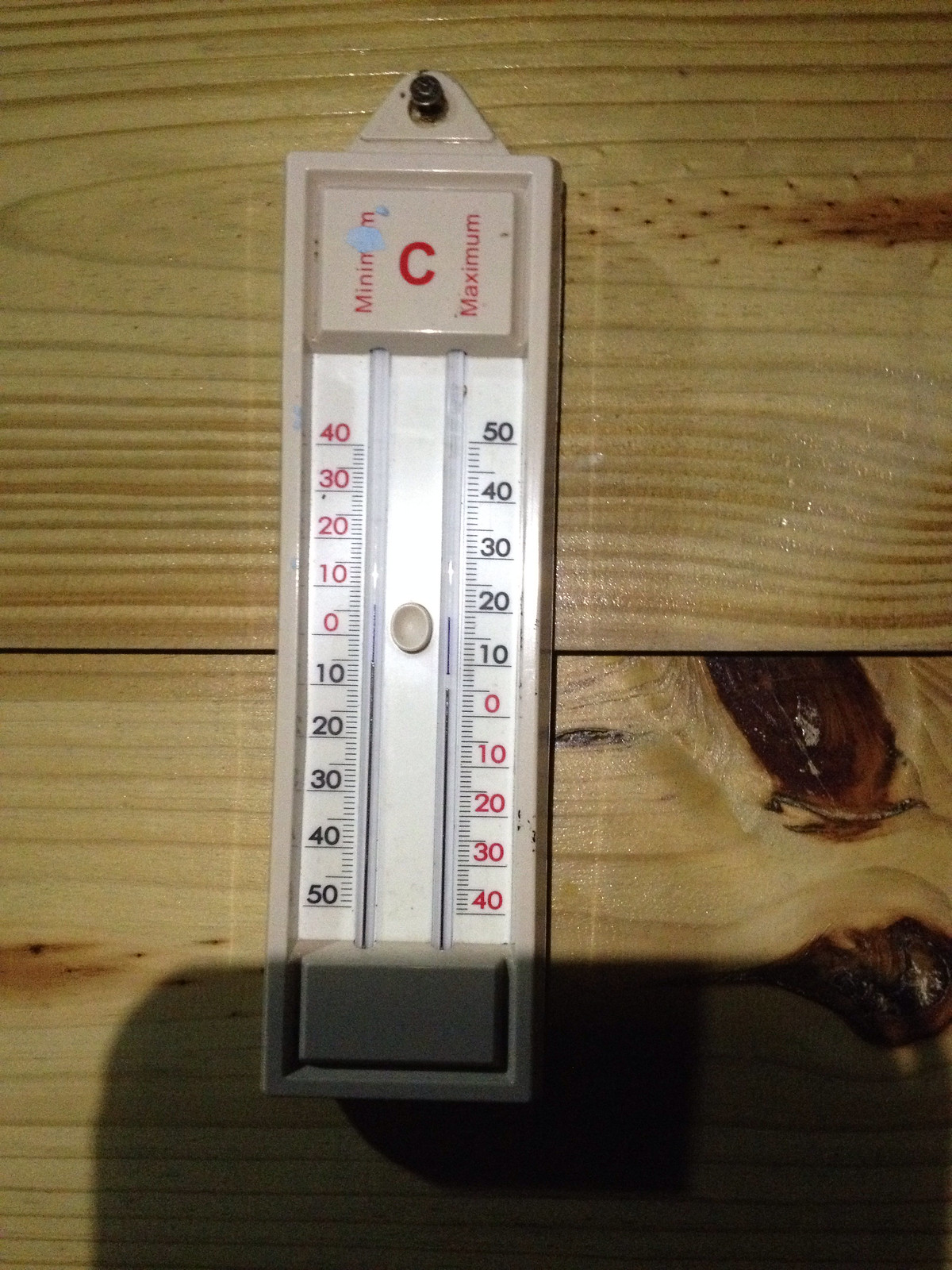The image features a pale, brownish-blonde wooden table as the background, heavily marked with various wood grains and brown gouges. A distinct cut divides the table horizontally almost at the center, creating two noticeable sections. There is an off-camera shadow adding an element of mystery, suggesting an unseen object.

Hanging on a black nail is a temperature gauge with a pale beige body, measuring degrees in Celsius. The gauge has two distinct scales: on the left, labeled "minimum," the scale ranges from -50 to +40, while on the right, labeled "maximum," it spans from -40 to +50. Both sides have numbers in red from -10 to 40, and in black from 0 to 50.

The gauge indicates the minimum temperature as 3 degrees Celsius and the maximum as 19 degrees Celsius. This suggests that the image, possibly taken in a workshop, monitors temperatures to ensure conditions remain within a specified range for optimal operation or storage.